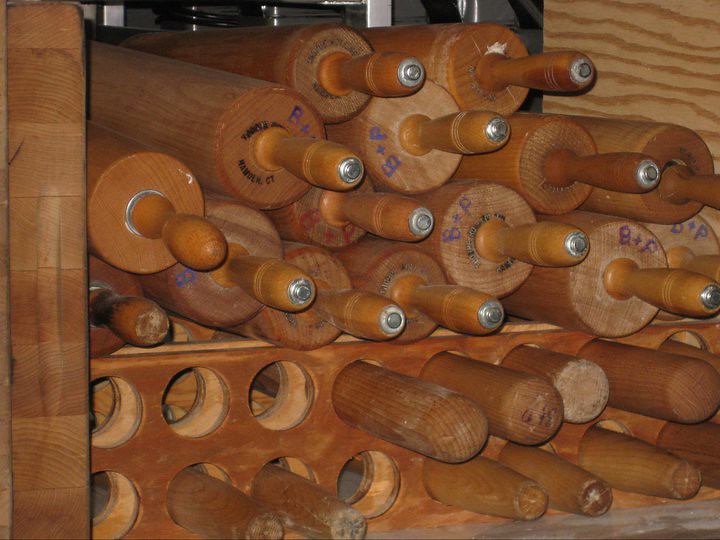The image is a detailed close-up photograph of a large, pyramid-shaped stack of wooden rolling pins, organized within a wooden rack. The primary focus is on two distinct types of rolling pins arranged in different tiers. 

At the top, there are 15 traditional wooden rolling pins, made of a dark brown to maple-colored wood, stacked haphazardly on top of each other. Each pin features handles, with most handles having a silver screw or metal cap at the very tip. Some of these rolling pins display the initials "B&P" written in purplish-blue marker on the ends, indicative of their use or ownership.

Below this pile, the rack consists of a wooden panel with round holes cut into it, hosting an array of 10 solid wood dowels used as rolling pins. These pins lack handles and are more uniform and narrow in design compared to those on the top shelf. The panel with holes is part of a structured wooden cupboard.

The backdrop of the image includes a vertical wooden section, possibly the edge of a cutting board, with additional wooden grains visible on the sides and a dark gray background beyond. This setting possibly suggests that the arrangement is located in a bakery or similar establishment.